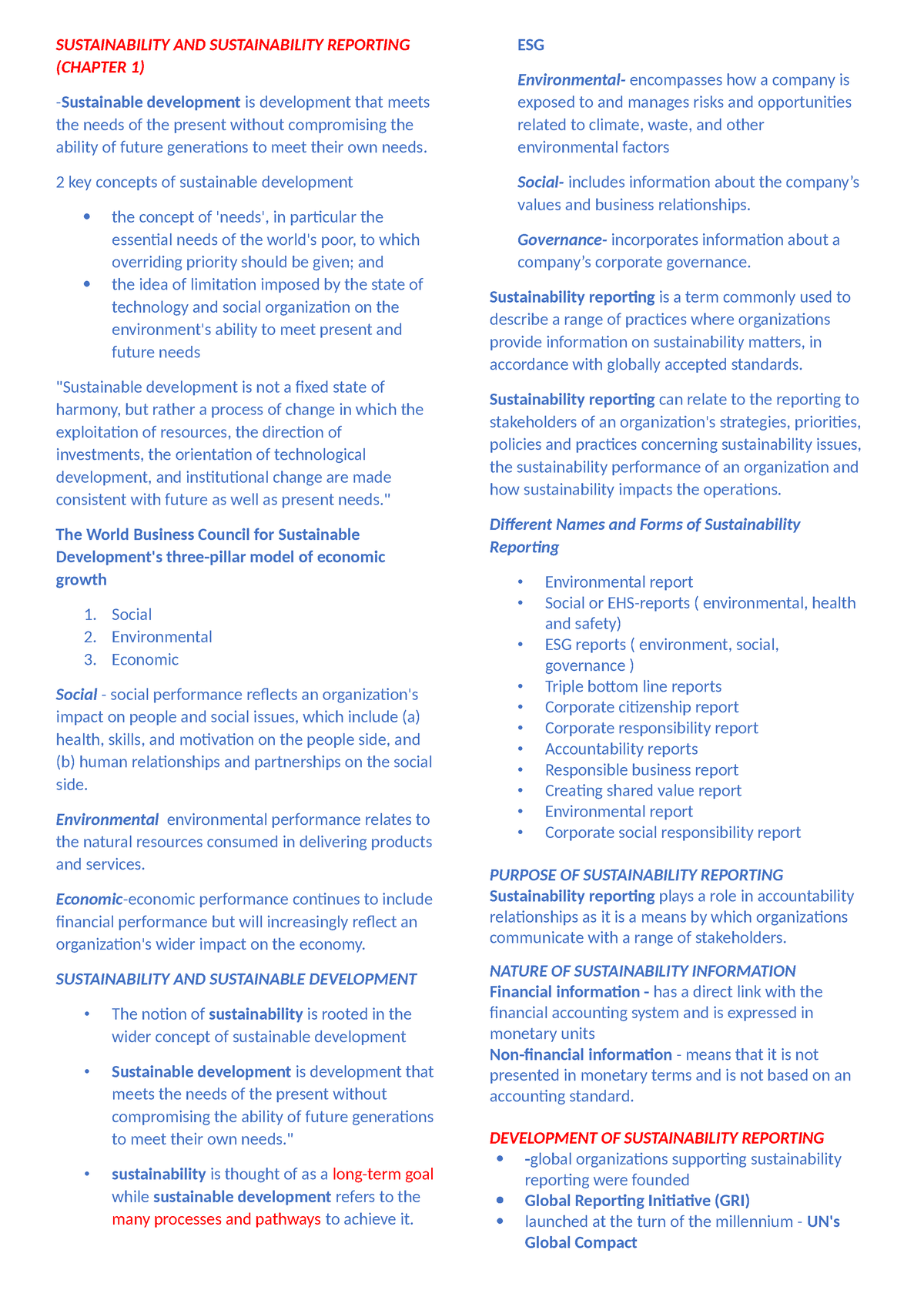This image is a screenshot from a website or possibly a scanned page from a book. The layout features a white background with primarily blue text, interspersed with a few red headers. There are two notable red headers and an additional red line. The main title, "Sustainability and Sustainability Reporting, Chapter 1," is positioned on the left side of the page and the content is structured into two columns.

In the first column, the section begins with the header "Sustainable Development," followed by a definition: "Sustainable Development is the development that meets the needs of the present without compromising the ability of future generations to meet their own needs." It highlights two key concepts of Sustainable Development, presented as bullet points. The text elaborates that Sustainable Development is not a fixed state of harmony, but a continuous process of change. This process involves the exploitation of resources, direction of investments, orientation of technological development, and institutional changes, all aimed at aligning with both current and future needs. This detailed explanation occupies several paragraphs and concludes the first column.

The second column starts with the header "ESG," which stands for Environmental, Social, and Governance. It contains individual sentences explaining each component of ESG. Following this, there are two more paragraphs discussing Sustainability Reporting in-depth. The section includes about a dozen bullet points, listing different names and forms of Sustainability Reporting. The column ends with a final header in red text, "Development of Sustainability Reporting," which is followed by two or three concluding bullet points. The content then comes to an end.